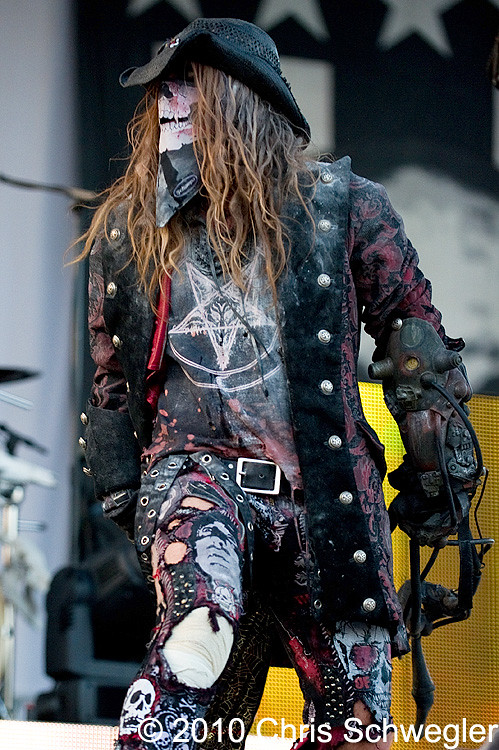The image shows a man dressed in an elaborate pirate costume standing outdoors in the middle of the day, possibly at a concert or similar event. He is positioned directly in the center of the image and is wearing a dark, leather pirate jacket adorned with various designs, topped with a hat and scarf. His outfit includes a colorful shirt and intricately painted pants featuring skull designs on both legs. He has long hair and a belt with a prominent buckle. 

In the background, there is a white wall adorned with a flag or large poster and possibly a screen, with musical instruments visible, hinting at a concert setting. The predominant colors in the image are black, white, gray, red, dark red, pink, maroon, silver, gold, yellow, and brown. 

In the bottom right corner, the text "Copyright 2010 Chris Schweigler" is visible. The man is caught in a mid-walking pose, looking off to the right side of the image, adding a dynamic element to the photograph.